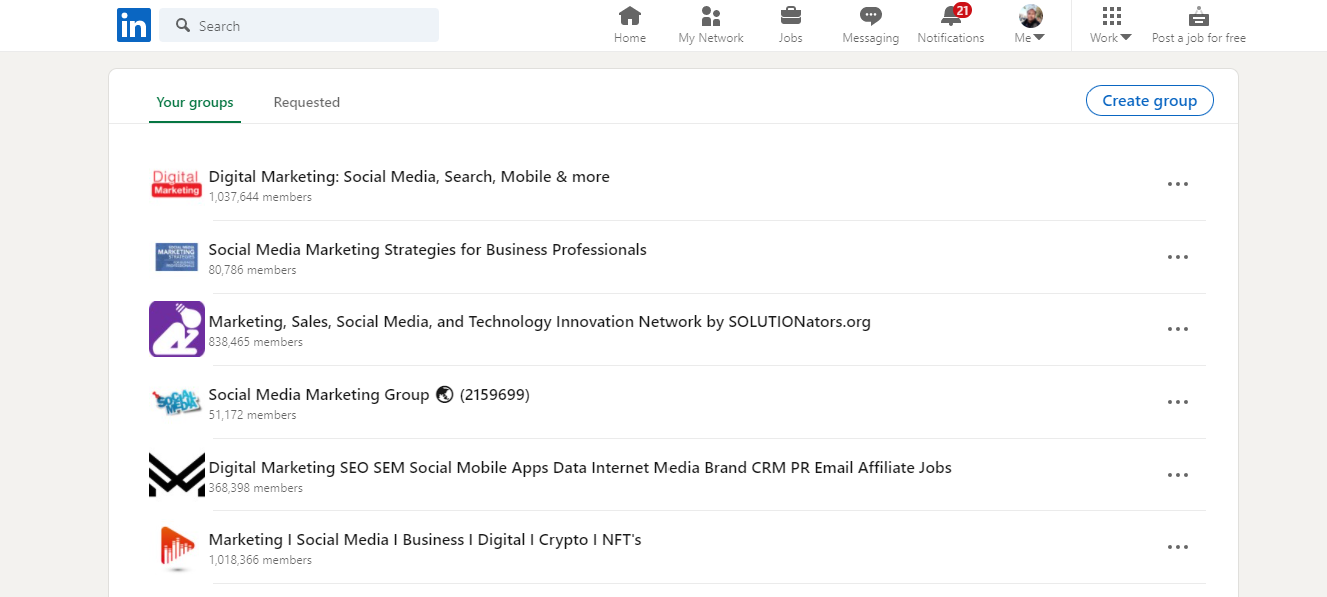The image has a gray background and prominently features a blue square with a white letter "N" in its center. Below this, there is a search bar accompanied by a magnifying glass icon. The top navigation bar displays several options: "Home," "My Network," "Jobs," "Messaging," and "Notifications," the latter of which has a red circle with the number "21" in white, indicating pending notifications. Additional options include "Me" and "Work."

The main section of the imagery consists of three rows, each containing three gray rectangles. One of the rectangles highlights an option to "Post a job for free." Another section invites users to explore "Your Groups," marked in green, with options such as "Requested" and "Create Group," the latter presented in a blue button-like oval. 

In another part of the image, a collection of topics like "Digital marketing," "Social media," "Search," "Mobile," and others are listed, accompanied by three horizontal dots, indicating additional options.

The description further touches on "Social media marketing strategies for business professionals" and lists relevant categories: "Marketing," "Sales," "Social Media," and "Technology Innovation Network." These categories are associated with a site named "Solution.org," where the word "Solution" is written in capital letters.

Additionally, the image features a "Social Media Marketing Group," marked by an icon of a globe and a parenthesis containing numbers, followed by three horizontal dots.